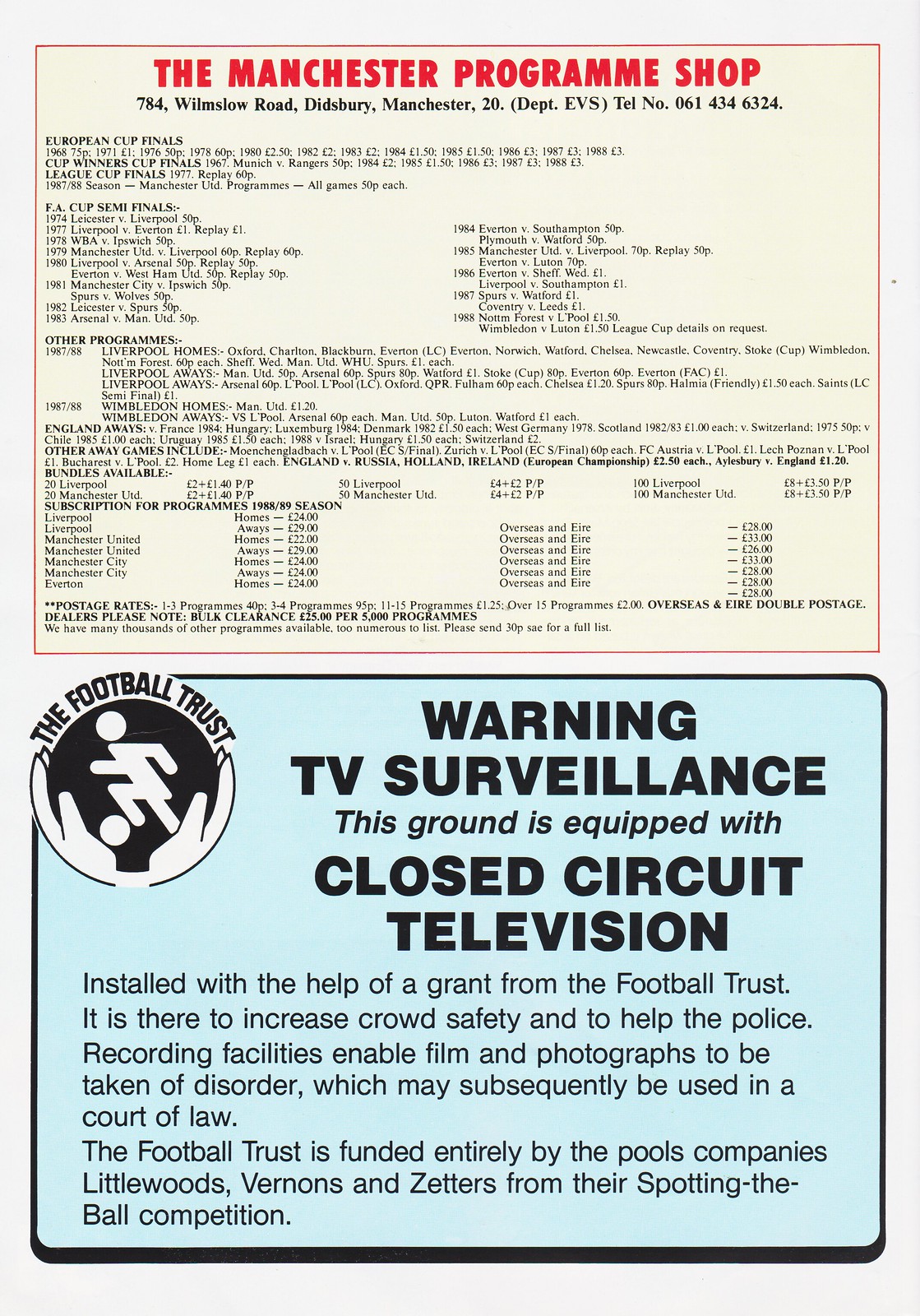This image features a detailed advertisement in landscape orientation for the Manchester Program Shop, prominently utilizing spot colors of red and light blue against a primarily white background. At the top, bold red lettering announces "The Manchester Program Shop," followed by the address "784 Winslow Road, Didsbury, Manchester 20," and the telephone number "061-434-6324." Below this information, several lines of text enumerate various soccer events such as European Cup Finals, Cup Winner Finals, League Cup Finals, and FA Cup Semifinals, along with other available programs.

The lower half of the advertisement is set on a light blue background bordered in black. In the top left corner of this section, a circular logo depicts two hands holding a caricature of a soccer player kicking a ball, encircled by the words "The Football Trust." To the right of the logo, the ad issues a warning in bold black text: "TV Surveillance. This ground is equipped with closed-circuit television." Beneath this warning, in smaller black text, is an explanation: "Installed with the help of a grant from The Football Trust, it is there to increase crowd safety and to help the police. Recording facilities enable film and photographs to be taken of disorder which may subsequently be used in a court of law." Further down, another paragraph emphasizes, "The Football Trust is funded entirely by the Pools Companies: Littlewoods, Vernons, and Zetters from their 'Spotting the Ball' competition."